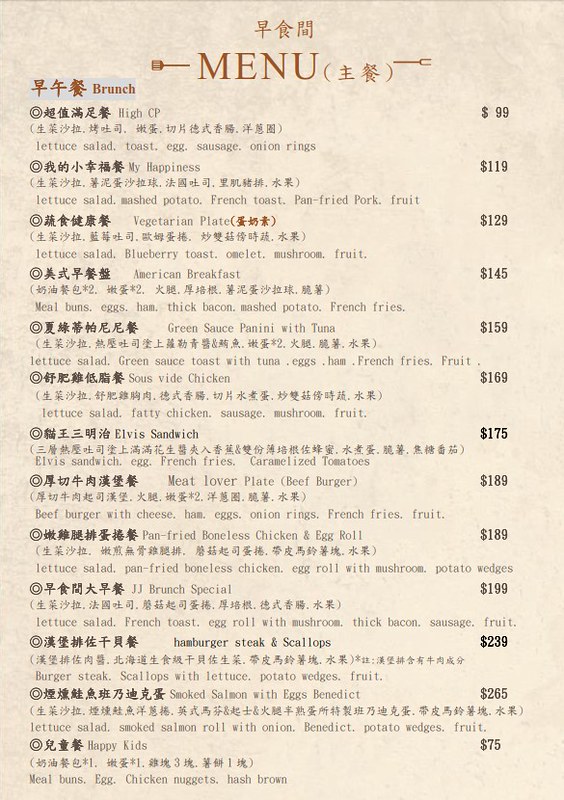This image features a menu, likely from a Chinese restaurant, characterized by its bilingual presentation of menu items in both Chinese (or possibly Japanese) and English. The menu has an off-white background, with the title at the top featuring text in Chinese (or Japanese) and the word "Menu," both printed in a reddish-orange ink. Below these titles, aligned to the extreme left, there is another Chinese or Japanese word presumed to signify "brunch," as it is accompanied by the English word "Brunch."

The menu lists various food items, each item paired with its price on the far right. For instance, the first item is listed as "High CP" and is priced at $99. Each menu item is prefaced by a small circle with an even smaller circle inside, serving as bullet points for the list. The overall layout and detailed bilingual description provide a clear view of the available brunch options and their costs.